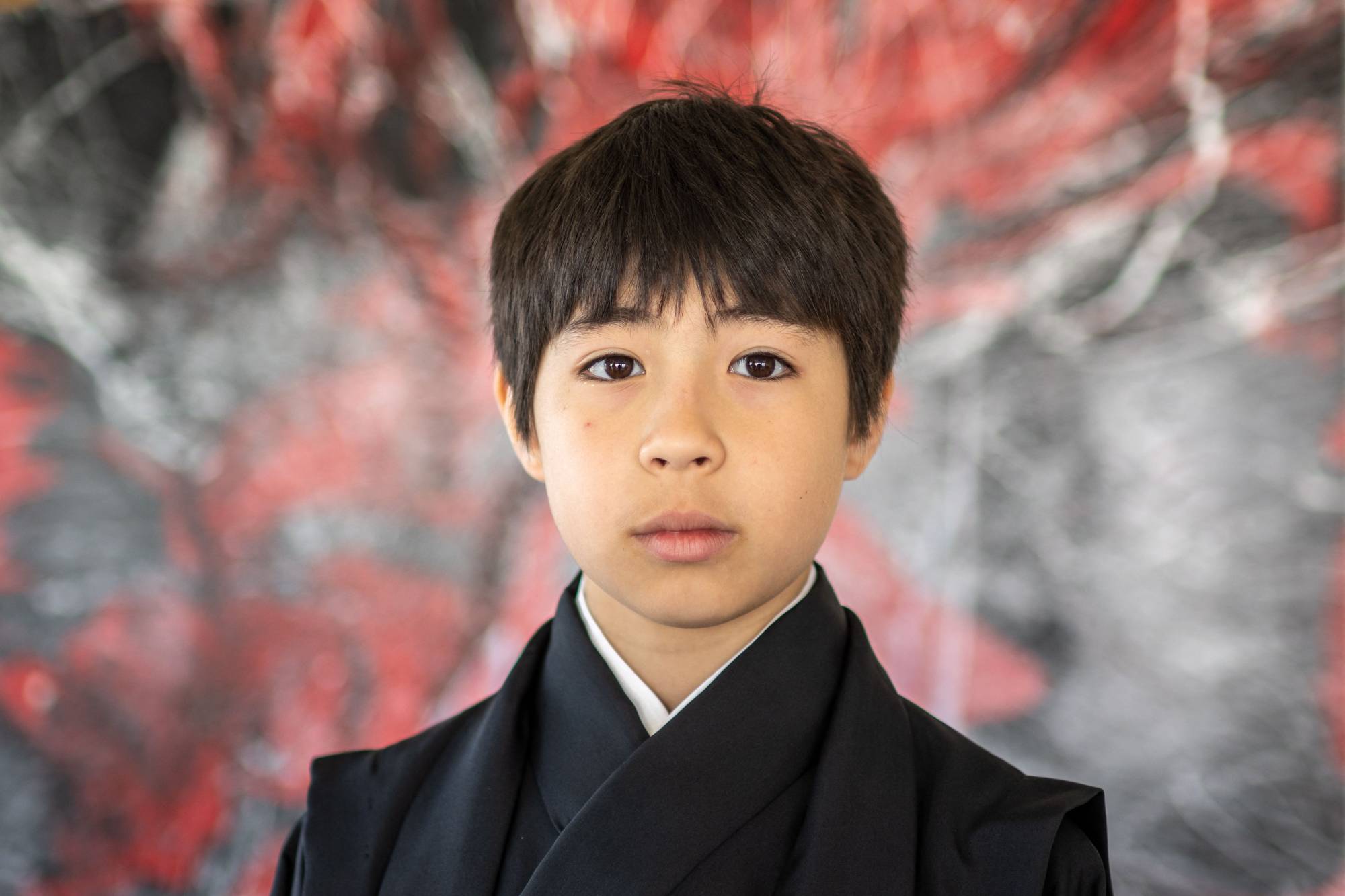In this detailed photograph, a young boy of Asian descent, appearing to be between 9 and 12 years old, is captured from the shoulders up. His thick, short dark hair frames a face with dark brown eyes and lightly tanned skin. He wears a formal black traditional garment, distinguished by a high collar and subtle white piping around the neck area. The boy's expression is neutral, not indicating any particular emotion. The background features an abstract design with shades of gray, red, and white, blurred to keep the focus on the boy. Overall, the image conveys a sense of calm and tradition, with no text present to provide additional context.